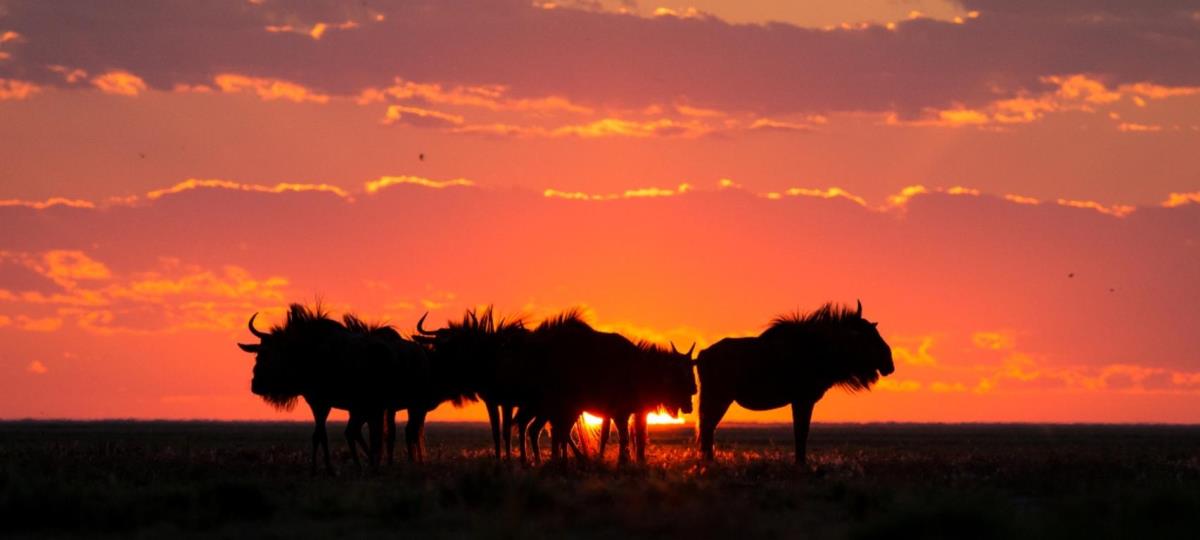The image portrays a breathtaking African prairie scene at sunset. The foreground features a close group of silhouetted wildebeests, their forms defined by the setting sun behind them. The intricate details reveal the animals’ long legs, heavy heads, and beards, with some showing distinct horns. There appear to be four or five wildebeests standing closely together, some facing right and others left, creating a picturesque herd pattern. The ground beneath them is dark, almost blending into the horizon. The sunset itself is a vibrant spectrum of purples, golds, oranges, and reds, casting a magnificent glow that gilds the edges of the scattered, puffy strata of clouds above. The sun, partially obscured, peeks through the legs of the wildebeests, adding a dramatic aura that enhances their silhouette against the richly colored sky.